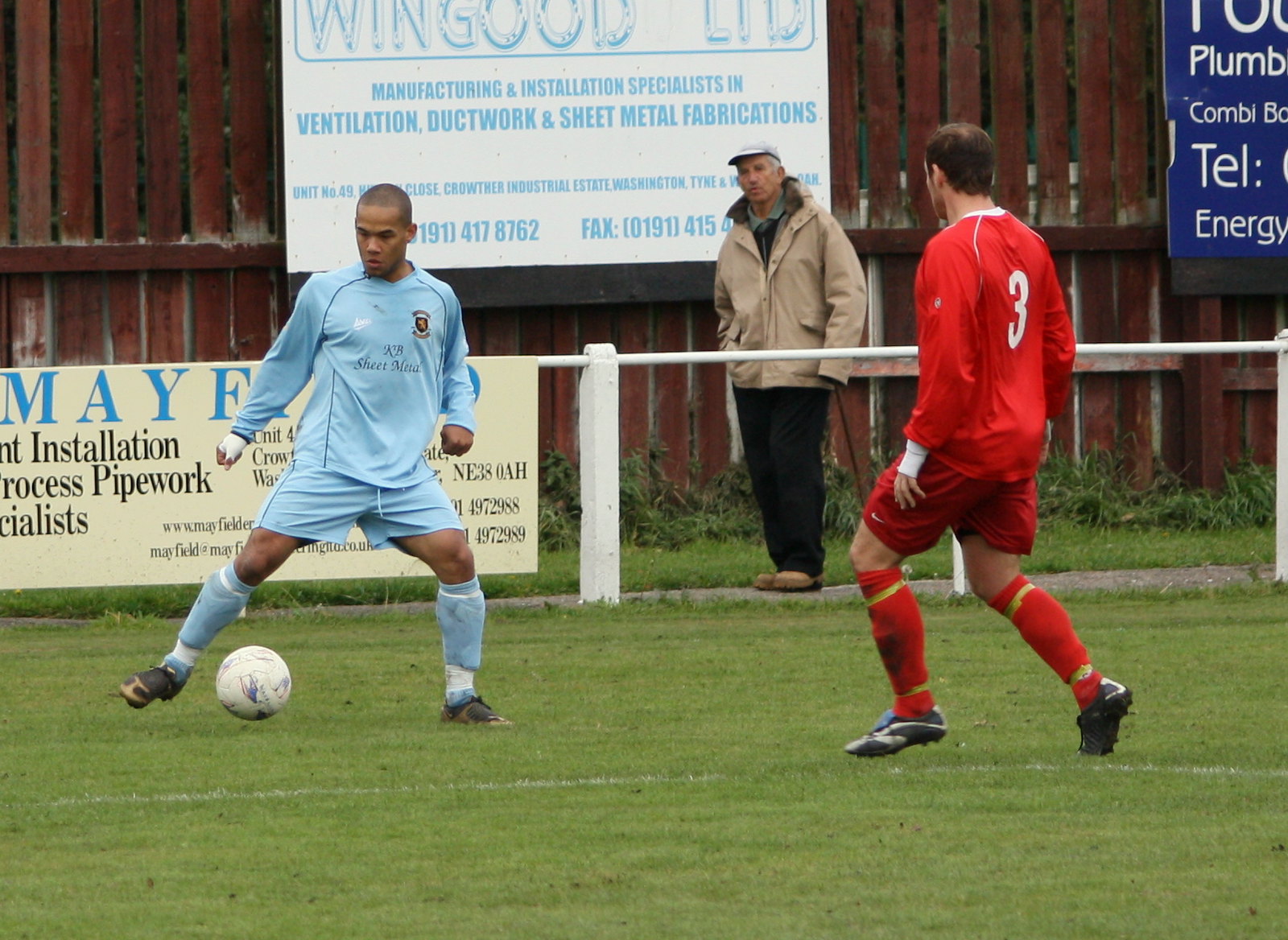The slightly out-of-focus full-color photograph captures an outdoor daytime soccer match. In the foreground, two players are in mid-action on a lush green field. The player facing the camera wears a light blue uniform of long sleeves, shorts, and socks, and is actively kicking a white soccer ball. Opposite him, with his back to the camera, stands player number three in a red uniform with red and yellow-trimmed socks; he appears to be slightly balding.

On the other side of the white fence surrounding the field is an older spectator, distinguishable in a tan jacket, dark pants, and a white cap. Several sponsor signs are affixed to the tall brown wooden fence in the background. The prominent white sign partially visible reads "Mayfield Installation Process Pipework Specialist," while another sign reads "Wingood Limited, Manufacturing and Installation Specialists in Ventilation, Ductwork, and Sheet Metal Fabrications." A blue sign indicating something related to plumbing is also discernible among the advertisements.